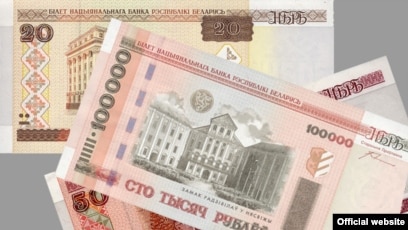The image features three distinct types of foreign currency bills, layered across each other in a landscape orientation. The top bill, angled slightly downward on the right-hand side, is a light pinkish color with shades of white. It prominently displays a large, hand-drawn building with huge columns in the center, and the denomination "100,000" on the left-hand corner. Below it, partially covered, is a reddish bill marked with the number "50." This bill, too, has an illustration of a building, though it is less visible due to the overlap. Towards the top left-hand side of the image lies a yellowish bill with hints of pink, showing a large building and the denomination "20" on its left side. The currencies, each featuring foreign characters, are set against a medium gray background.